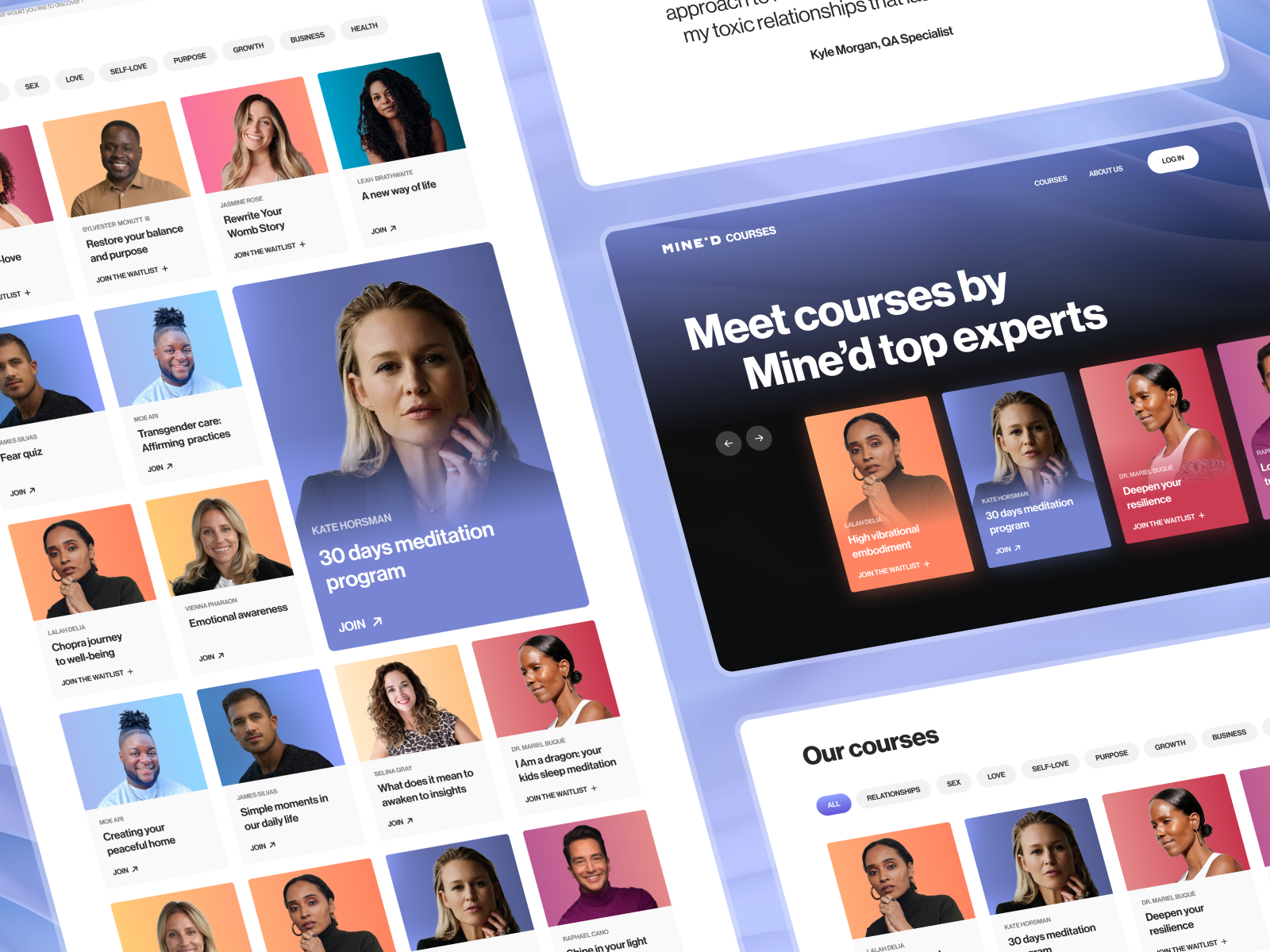This image appears to be an advertisement arranged diagonally. On the left side, there is a gallery featuring an assortment of headshots of men and women, each headshot set against a uniquely colored background. Moving to the right side, there are several partial screenshots of web pages. The central screenshot stands out with a dark black background and the text "Meet Courses by Mind Top Experts." Similar headshots of people against plain-colored backgrounds can be seen here as well. Below this is another section titled "Our Courses." At the very top, there is a fragment of another page containing part of a quote, though the entire quote is not visible due to the cropping of the image.